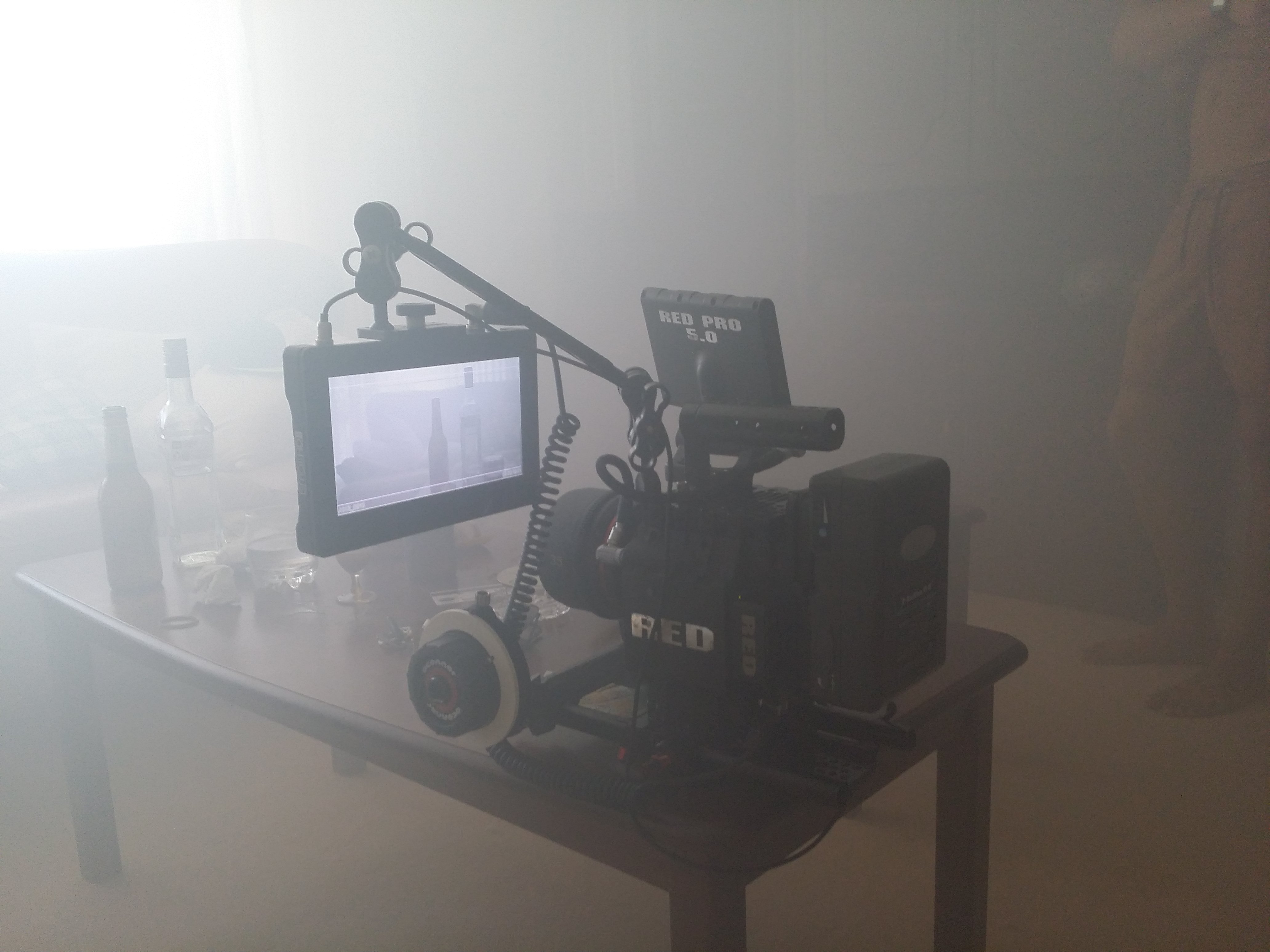In a hazy, smoke-filled room, a detailed photograph captures a sophisticated cinematography camera setup, prominently labeled with "Red" and "Red Pro 5.0". The black apparatus, positioned on a wooden table, features several moving parts, including a boom arm with an attached video monitor. The monitor displays the live feed from the camera, showing two alcoholic beverage bottles and assorted glasses on the table directly in front of it. Multiple cords connect the monitor back to the base of the unit, suggesting a highly professional setup. The table also holds bits of trash, further adding to the scene's cluttered appearance. To the right, partly obscured by smoke, stands a barefoot man wearing a wristwatch, though his face is not visible. The photograph conveys a sense of meticulous detail and complex equipment amidst the room's chaotic, hazy atmosphere.